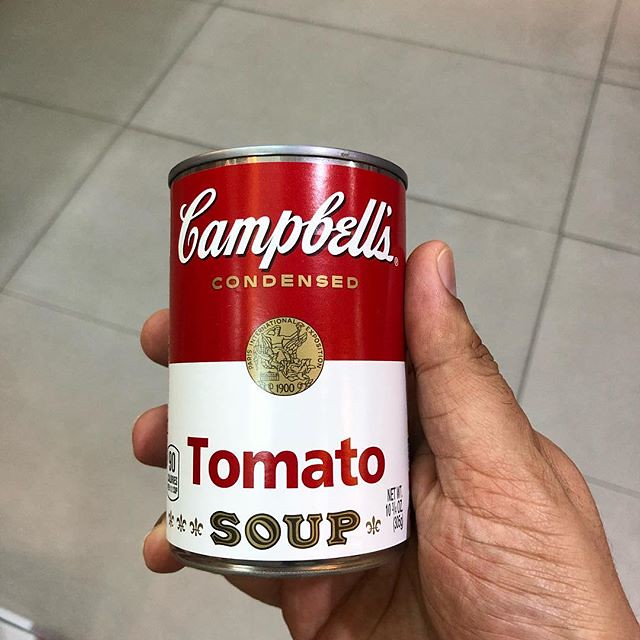In the photograph, an adult individual holds a single can of Campbell's Condensed Tomato Soup in their right hand. The classic Campbell's label is prominently displayed, featuring the distinctive red and white design. The word "condensed" is printed in gold script near the top of the label, while a small circular brand logo is situated above it. The word "tomato" is displayed in red against a white background toward the lower center of the label, with the word "soup" written in golden letters outlined in black. The hands grasping the can have very short nails and appear to belong to an Asian or caramel-colored individual, though it is difficult to discern their gender. The photograph is taken at an angle above a floor, which is adorned with gray rectangular tiles, providing a neutral background for the vividly colored soup can.